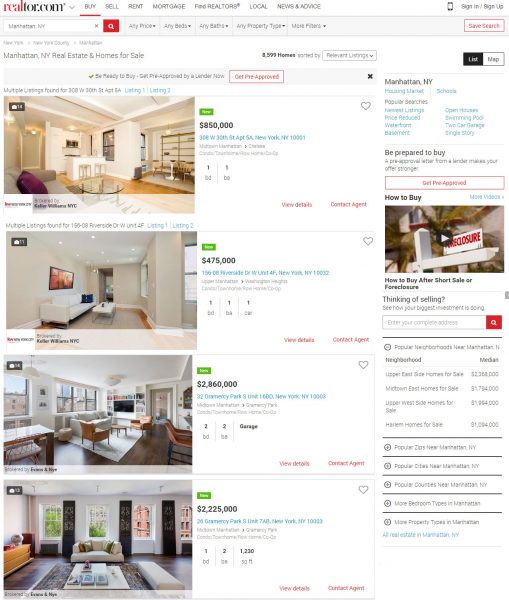The image depicts a page from Realtor.com, characterized by its distinctive color scheme with "Realtor" in red and ".com" in black against a predominantly white background. The site's interface is populated with a variety of navigation links at the top, such as "Buy," "Sell," "Rent," "Mortgage," "Find Realtor," "Local News and Advice," and a "Sign In/Sign Up" option located in the top right corner.

The page showcases a search for Manhattan, New York, revealing four property listings available for sale. These listings feature small, hard-to-read text but display varying price points: $150,000, $475,000, $2.8 million, and $2.2 million. The listings focus on interior shots, though it is unclear whether they depict houses or apartments due to the text size.

To the right of the listings, there is a video titled "How to Buy After a Short Sale or Foreclosure," offering guidance on related real estate processes.